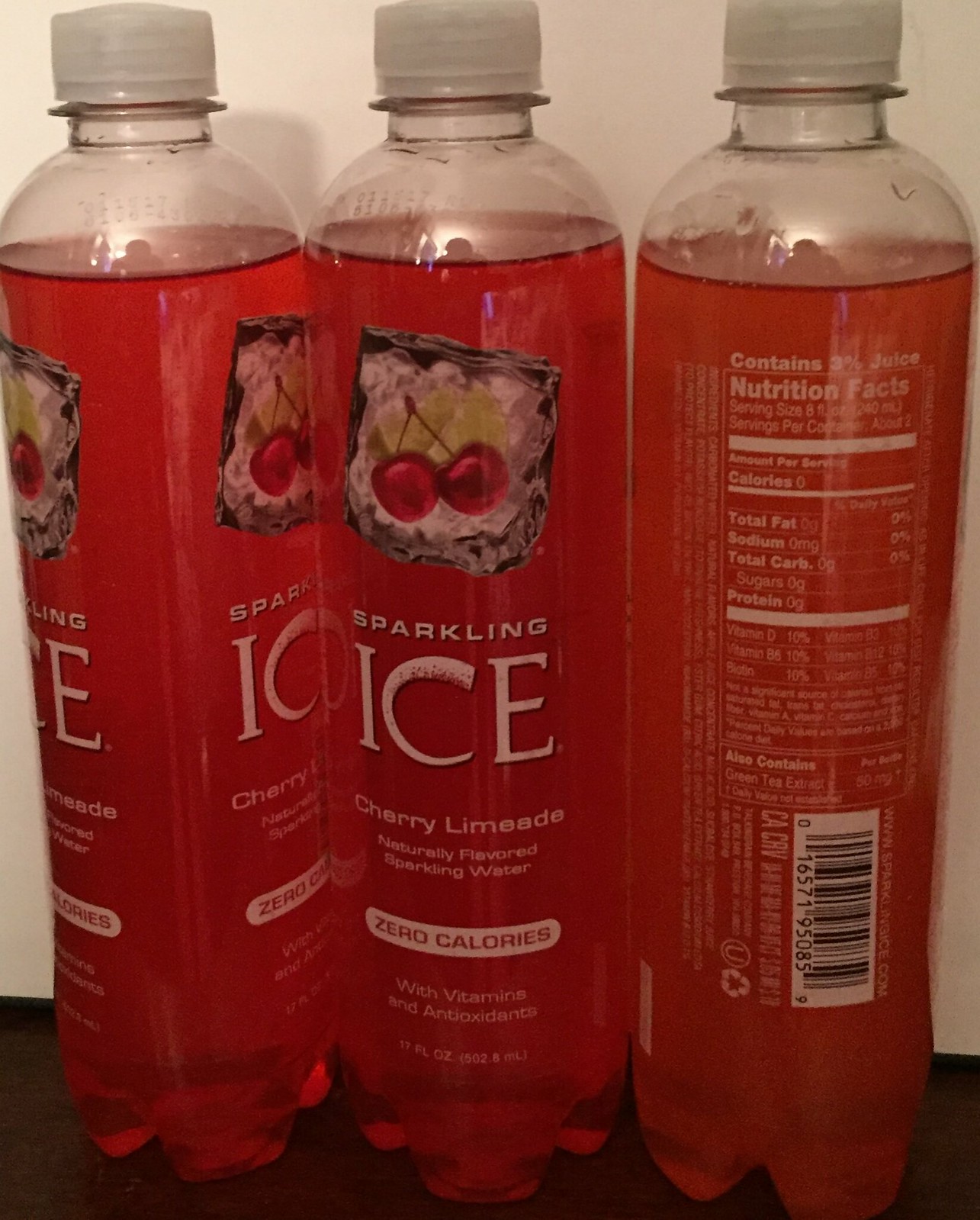In the image, a light gray wall serves as a minimalist background, complementing a smooth brown surface that could either be a floor or a table. Placed centrally on this surface are three identical bottles of a beverage called "Sparkling Ice." Each bottle is made from clear plastic, revealing a vibrant pink liquid inside, and is capped with a white top. The bold, white lettering of "Sparkling Ice" prominently displays the brand name.

The labeling on each bottle depicts a small, enticing basket filled with ripe cherries and fresh limes, illustrating the drink's flavor: Cherry Limeade. Beneath this image, the label notes a key selling point, "zero calories," emphasizing the drink's healthful appeal as a flavorful yet calorie-free sparkling water option.